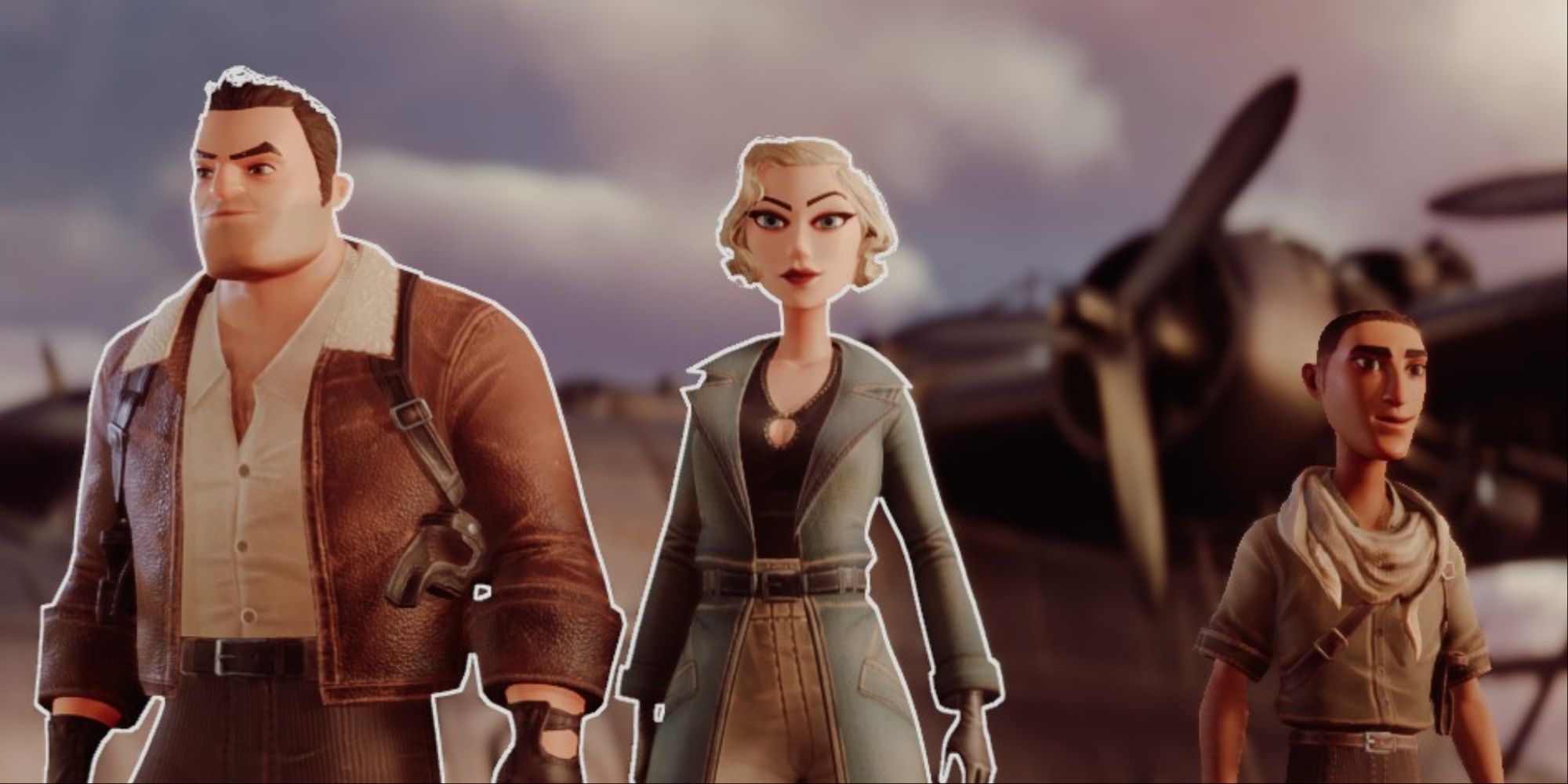The image features three AI-generated, semi-realistic characters standing in the foreground, all facing forward, with a cloudy sky and a muted, old-time airplane propeller visible in the background. On the left is a muscular man with short dark brown hair and an exaggerated jawline, dressed in a brown leather jacket, beige shirt, and brown pants. He is also wearing leather gloves and has two guns in holsters under his arms. Next to him in the center is a woman with chin-length blonde hair, light skin, and a long, bluish-grey trench coat cinched with a brown leather belt. She has a black top underneath and light greyish-brown pants. To the far right stands a younger male character with very short black hair, clad in a short-sleeved light brown shirt, brown pants, and an off-white scarf around his neck. The man and woman are depicted only up to their waist or thighs, while the younger character is shown to the waist. They are under the wing of a vintage airplane, adding a nostalgic element to the scene.